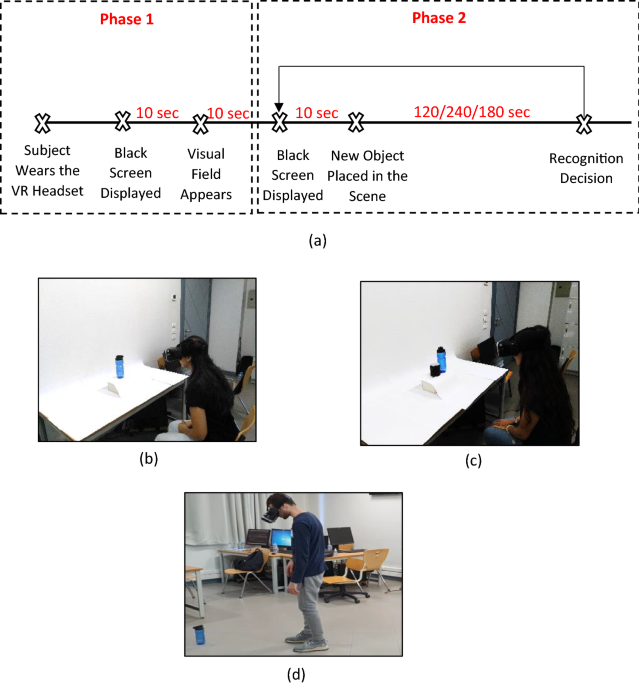The image portrays a comprehensive experimental setup involving virtual reality (VR) to test object recognition. At the top, it features two diagrams outlined with dotted dashed rectangles, representing Phase 1 and Phase 2 of the experiment, labeled as part A. Phase 1 shows a timeline where the subject wears the VR headset, followed by a black screen display, and then a visual field appears, with 10-second intervals marked by X's. Phase 2 continues with a black screen display, another 10-second interval, and the introduction of a new object in the scene, followed by a 120/240/180-second interval, concluding with a recognition decision.

Below the diagrams are three photographs labeled B, C, and D. Picture B and C show a woman wearing a VR headset, seated in front of a table, looking towards a wall, indicating different stages of visual engagement. Picture D depicts a man, also wearing a VR headset, standing and looking downwards, possibly in a classroom or laboratory setting. Each element of the image provides a detailed insight into the phases and execution of the VR-based object recognition experiment.